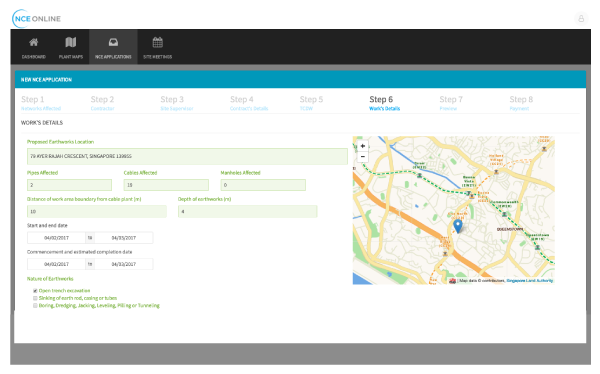The image displays a detailed view of a webpage layout centered around a map feature. In the top left corner, there is a distinct logo. Beneath this logo, a sleek black navigation bar spans horizontally, adorned with four icons; the third icon is highlighted by a subtle light gray background, indicating its active status. The main body of the page is set against a neutral gray background. At the very top of this section, a bold blue rectangle houses the title of the page.

Directly below the title, there is a secondary navigation bar labeled 'Step 1' through 'Step 8', with 'Step 6' clearly selected. Following this, the central feature of the page is a form, where the text fields are highlighted in green and the boxes themselves are set against a light green background for emphasis. Toward the lower part of the form, two sections contain two boxes each, marked by contrasting black text on white backgrounds, providing structured input areas.

Flanking the right side of the page, an interactive map stands out, depicting a dotted green line traversing diagonally from the top-left corner to the bottom-right corner. This line connects multiple points, each distinctly labeled, illustrating a path or route with relevant details. The visual composition effectively guides the user's attention from the navigation elements to the central interactive and input components.